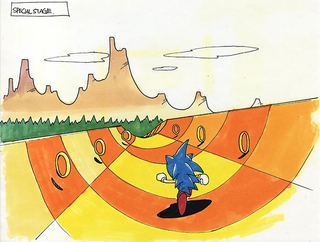The image depicts a colorful, cartoon drawing titled "Special Stage" in the top left. It features Sonic the Hedgehog running down the center of a highly stylized, orange and yellow checkered half-pipe. Sonic is shown from the back, mid-run, with his trademark spiky blue hair and white gloved hands visible. Surrounding the pathway are golden rings scattered along the sides, suggesting a typical collectible element from the games. On each side of the half-pipe, the walls rise in a pattern of orange and dark orange squares. In the background, lush green trees dot the landscape, leading to rugged, canyon-like mountains in the far distance. The sky above is a clean white with a few sparse clouds, emphasizing the contrast and vibrant colors of the scene. Sonic appears determined as he sprints forward, completely engrossed in his high-speed run.